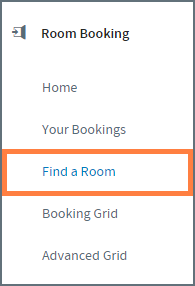The image depicts a small screen, likely from a mobile phone, featuring a user interface for a room booking application. The screen is framed by a thin dark gray border. The interface is set against a white background. At the top, there is an icon of an open door with an arrow pointing inward, suggesting an entry or access point. Accompanying this icon is the bold, black text "Room Booking."

Below the header, several options are listed in an indented format without accompanying icons, which could enhance the visual appeal. These options are:

1. **Home** - displayed in a gray font.
2. **Your Bookings** - also in a gray font, positioned with some vertical spacing below the Home option.
3. **Find a Room** - this option is highlighted with an orange selection indicator and is rendered in blue, showing either a cursor hover or a clicked state.
4. **Booking Grid** - shown in a gray font.
5. **Advanced Grid** - similarly displayed in a gray font.

Overall, the interface appears utilitarian and could benefit from additional visual elements to make it more engaging.